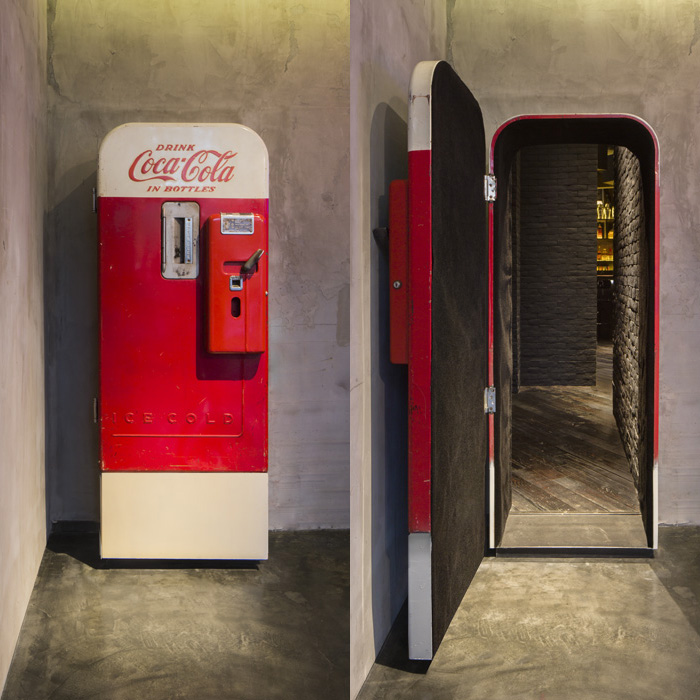The image consists of two juxtaposed panels that together reveal a fascinating interior feature. The left panel depicts what appears to be a vintage Coca-Cola vending machine door. This door, rectangular with rounded corners, prominently features a classic design with white and red colors. It bears the iconic slogan "Drink Coca-Cola in Bottles" in red cursive at the top. Below, there is an embossed label "ICE COLD" on the red portion, and a compartment where bottles would be dispensed. The walls surrounding this door are rough cement, contrasting with a darker gray concrete floor, adding to the vintage industrial ambiance.

On transitioning to the right panel, the previously closed Coca-Cola machine door is now open, unveiling a hidden entryway to a private bar. The interior space is inviting, with warmly lit shelving that holds glasses and bottles, lending a cozy ambiance. The floor transitions from the concrete exterior to light-gray brown diagonally laid hardwood. The walls inside are brick, painted gray, and contribute to the secluded, speakeasy-like atmosphere. This clever design invites curiosity and a desire to step inside and explore the hidden bar beyond the vintage facade.